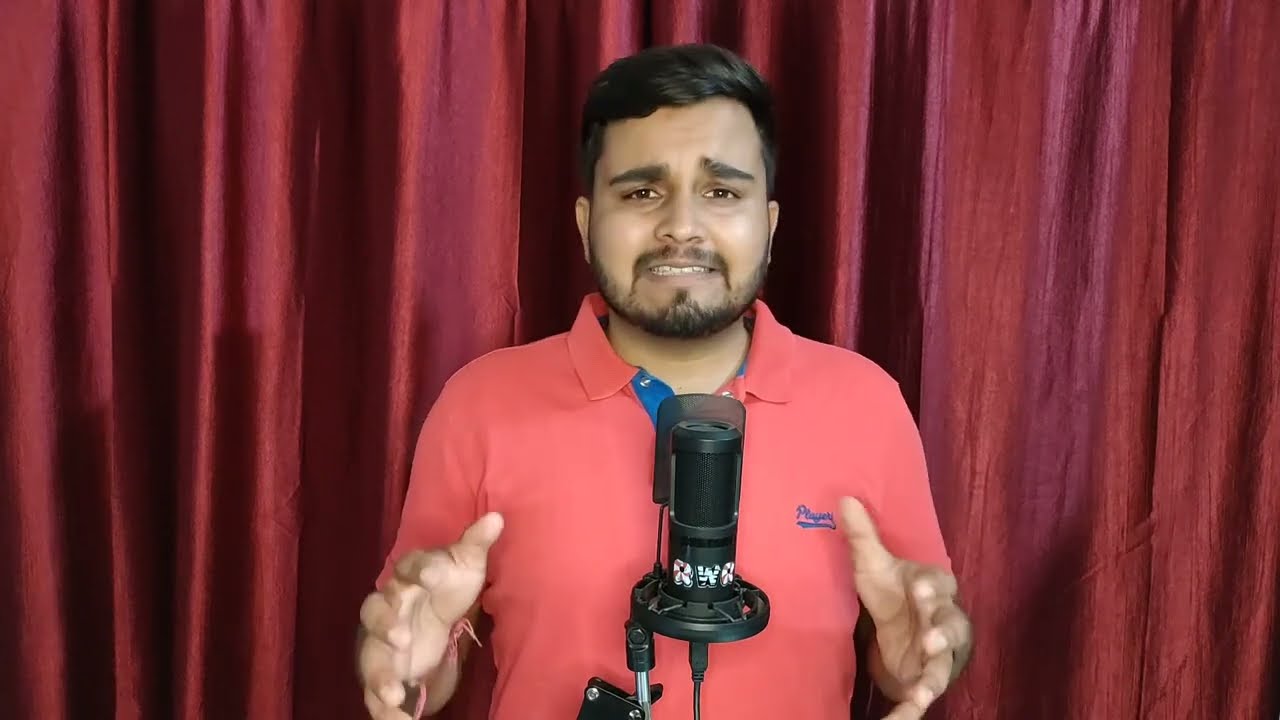The photograph features a bearded gentleman with cropped black hair styled to the side, standing about waist-up and staring intently into the camera. He is dressed in a light reddish-orange polo shirt adorned with a blue stripe down the center and a logo reading "PLAYERS" on the chest. The shirt also features blue detailing on the buttons. The man, who appears to be of Indian descent, is speaking into a black cylindrical microphone mounted on a stand labeled with the letters "R.W.R." His mouth is slightly open, his left eyebrow raised, and his eyes are squinted, conveying an expression of urgency or importance. He is actively gesticulating with both hands around the microphone, emphasizing his speech as though communicating something critical to his audience. In the background, there is an image of metallic-looking, maroon and black curtains, which creates a dramatic, glossy backdrop. The entirety of the scene is captured with a clear focus on the man's expressive gestures and earnest demeanor.